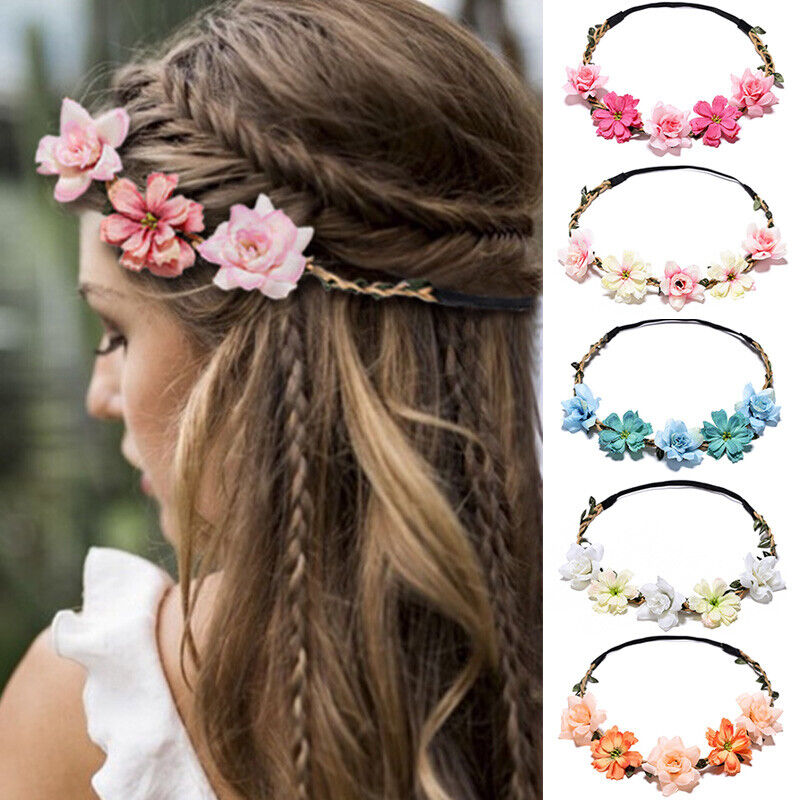The photograph captures a young woman with light skin and long, brown, curly hair accentuated with blonde highlights, elaborately braided and adorned with a vibrant floral headband. Part of her face is visible in profile as she gazes to her left. She wears a white, frilly shoulder strap, suggesting an elegant outfit. The headband features a striking arrangement of three pink flowers interwoven with brown vine-like bands. 

Occupying the right-hand side of the image, against a blank white background, are five similar floral headbands, each decorated with differently colored flowers: a combination of dark and light pink, white and pink, blue and teal, white and yellow, and a blend of orange hues. The overall composition suggests an advertisement for these beautifully crafted headbands.